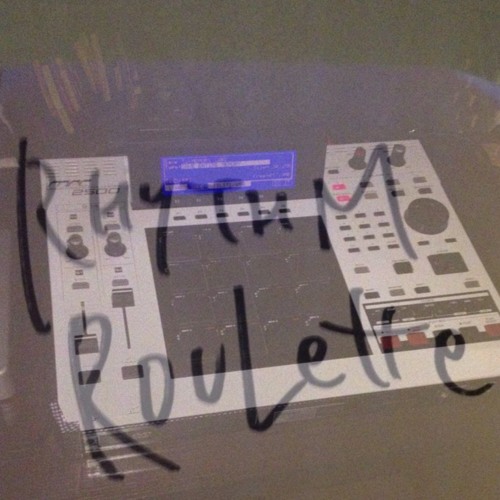The image features a white rectangular device, likely a drum machine, prominently labeled "Rhythm Roulette" across the top in black text. The device's central portion consists of a black square filled with small pads, suggesting it can assign percussive elements, which reinforces its identity as a drum machine. At the top, a small blue screen displays text, surrounded by various buttons and knobs. On the left side, there are two black knobs, sliding levers, and possible outlet areas. The right side hosts a large black dial, two red buttons, and numerous smaller buttons. The background is indistinct due to the blurry, washed-out contrast, making the edges of the device less clear, but the general layout suggests a sophisticated electronic control interface under a dim overlay.